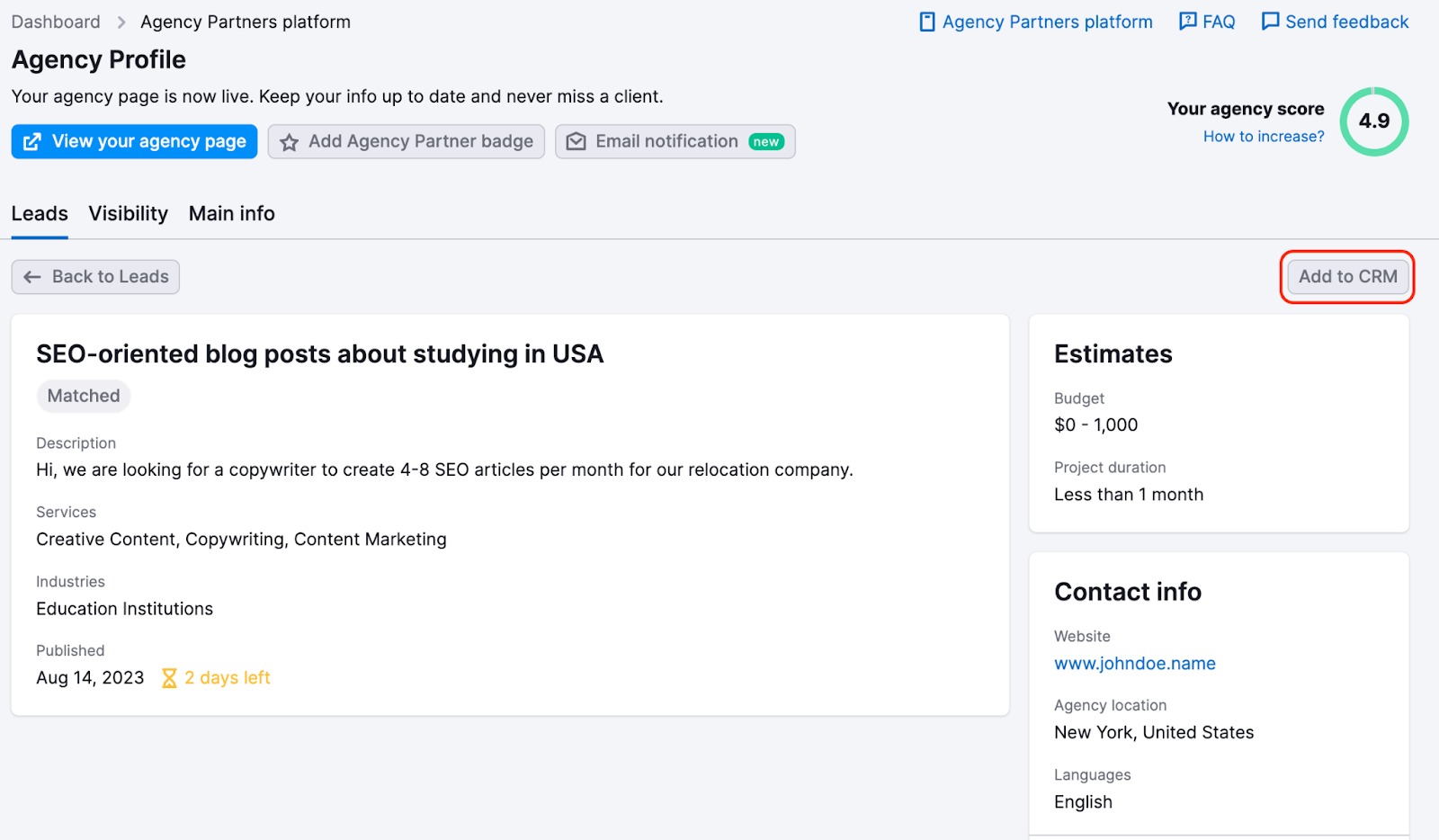A screenshot captured from a computer screen shows a website with a background in a faint grayish-blue tint. The webpage is predominantly structured with white rectangular sections. At the top, the navigation bar features the title "Dashboard" followed by an arrow pointing to "Agency Partners Platform." The top bar is highlighted in blue and contains links labeled "Agency Partners Platform," "FAQ," and "Send Feedback."

On the left side, in black text, a prompt reads, "Your agency page is now live. Keep your info up to date and never miss a client." Below this text, there are several clickable rectangular buttons—one saying "View Your Agency Page", another labeled as "Add Agency Partner Badge", and a third option titled "Email Notification" with a small green circle denoting it as "New."

Towards the bottom of the screen, sections are labeled "Leads," "Visibility," and "Main Information." On the right-hand side of the page, an indicator showcases "Your Agency Score: 4.9" with an adjacent link, "How to increase." A button to "Add to CRM" is prominently outlined with a red rectangular border.